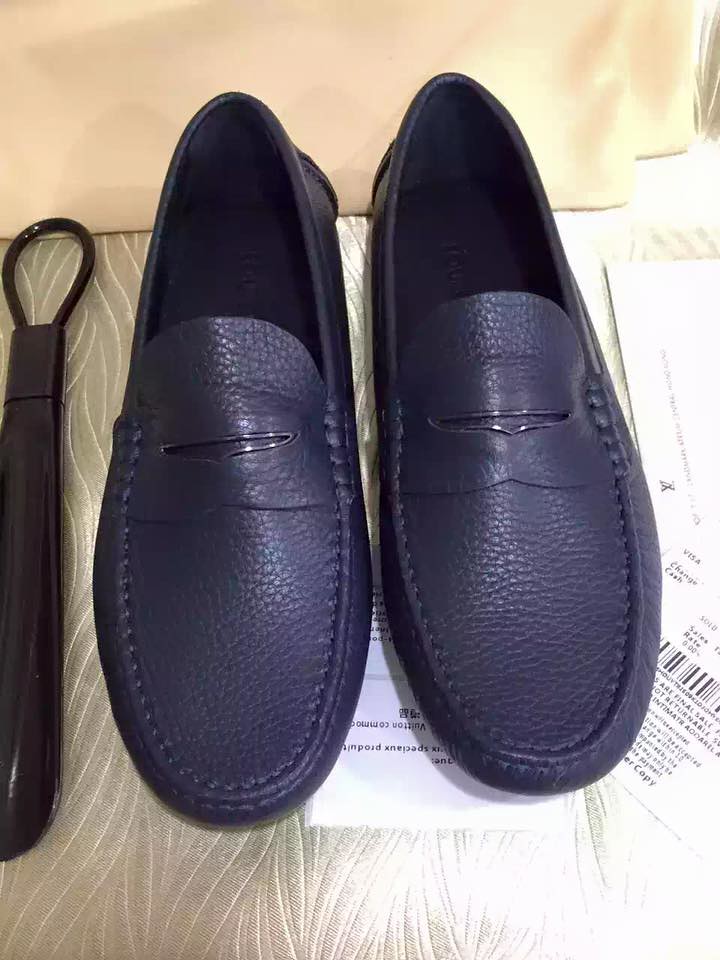The image depicts a close-up of a pair of penny loafer style shoes positioned with their toes facing the viewer and their heels towards the background. The shoes are made of leather and feature intricate stitching and a design on the top, with their deep purple color appearing almost black. They rest on a silvery, shiny, and patterned fabric surface. To the left of the shoes is a shoe horn, which is brown with a circular hook at the top and a textured, cotton-like material at the bottom. On the right side of the image, and underneath the shoes, are white sheets of paper with black writing, although the text is blurred. The background features a light brown curtain.